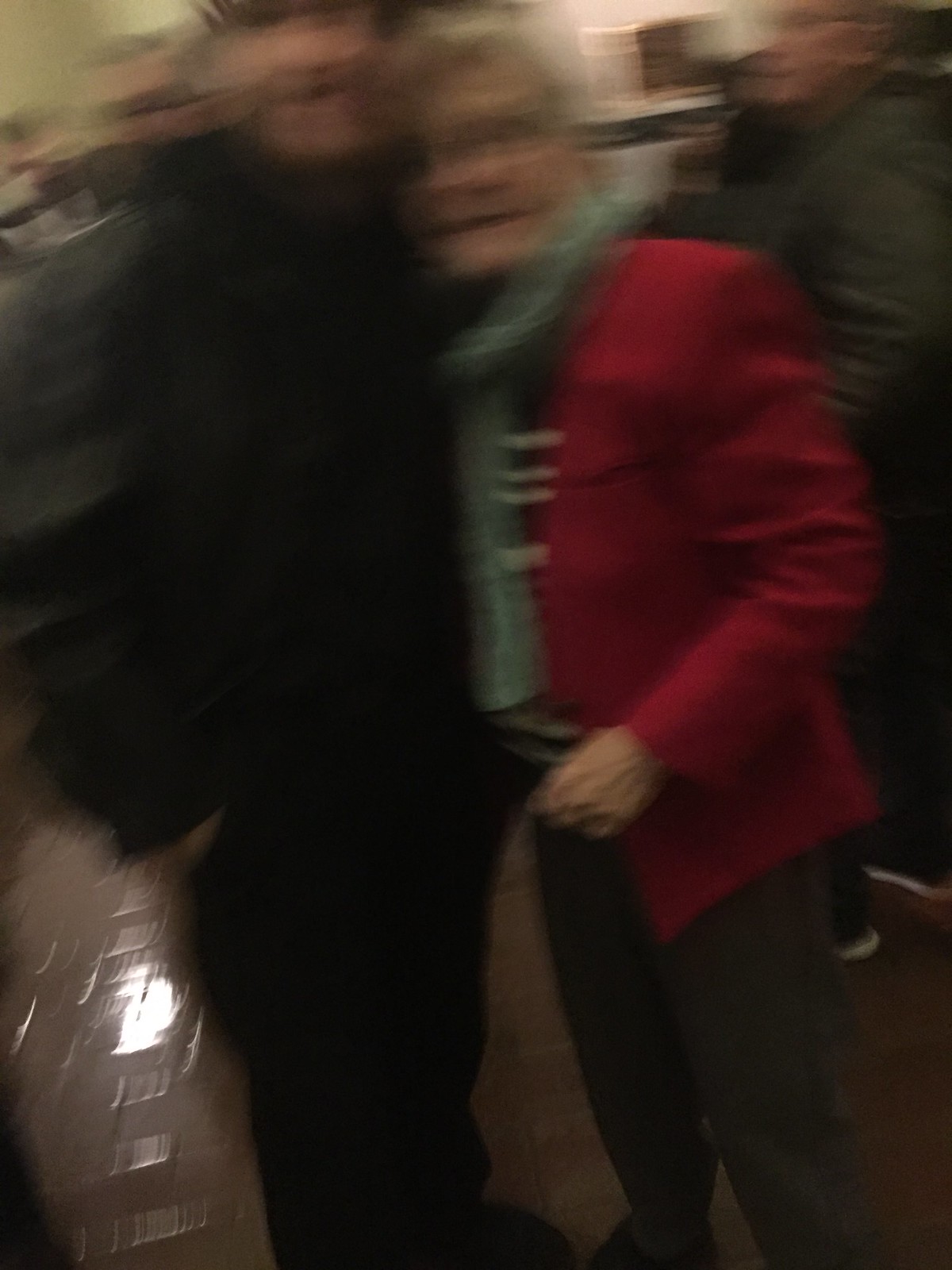This extremely blurry color photograph depicts two people standing in the foreground, seemingly posing for a picture. The person on the left, who appears to be a man, is dressed in dark clothes, including a dark jacket, black pants, and black shoes. There is a clear, reflective object near his leg on the left side of the image. The person on the right is an older woman, wearing a red jacket, a green scarf, and dark gray pants. She appears to be leaning against the man. Both individuals are possibly smiling, though facial details are indiscernible due to the blurriness. Behind them, a person in a green jacket, along with other indistinct figures, can be seen standing on a shiny brown floor indoors. The photograph is devoid of any legible writing, plants, flowers, trees, or animals.